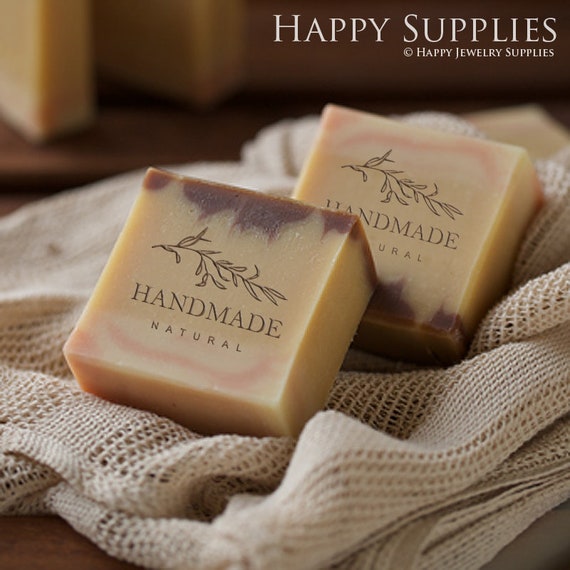This image captures a detailed and aesthetically pleasing scene featuring two square-shaped bars of handmade soap, nestled in an open weave tan fabric that rests upon a brown wooden surface. Each soap bar is beige with an ombre effect, transitioning to a darker brown on one end, and they feature a brown image of a leafy branch underneath which reads "handmade natural." In the background, there is a wooden shelf with additional bars of soap standing on it, though they are out of focus. The cloth beneath the soaps is tan, and light is illuminating the scene from the left, adding warmth and highlighting the natural, artisanal quality of the soaps. In the upper right-hand corner, the inscription "happy supplies, copyright, happy jewelry supplies" is subtly visible. The overall composition emphasizes the handcrafted, natural essence of these soaps.